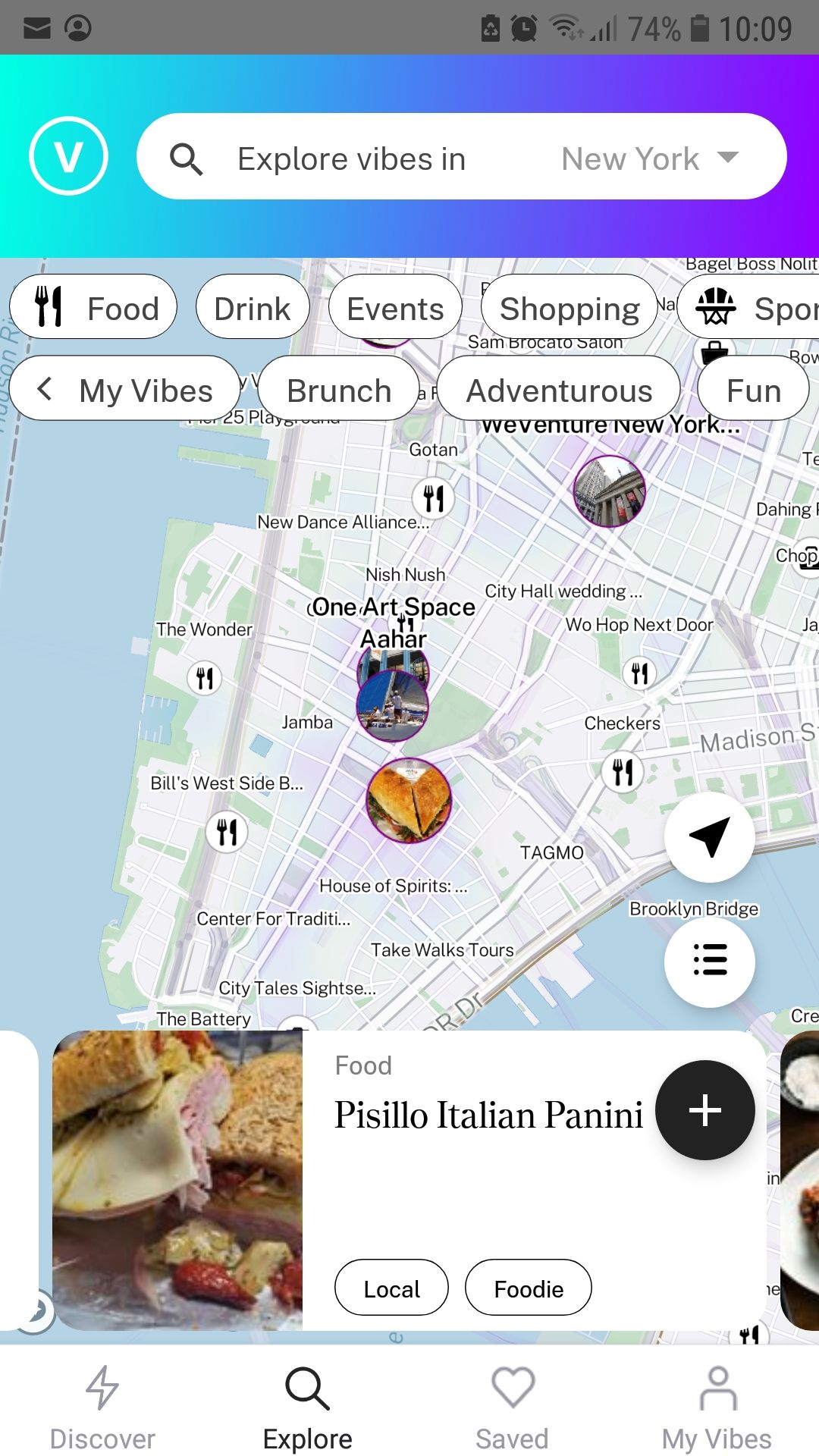A cell phone screen displays a vibrant, user-friendly interface geared towards food exploration. At the top of the screen, there is a gray status bar featuring an envelope icon and a person profile icon on the left. On the right, the bar shows a battery icon indicating 74% charge, an alarm icon, Wi-Fi signal bars, and the time, 10:07.

Beneath the status bar, a gradient field transitions from bright turquoise-green on the left, through blue, to purple on the right. Within this field, a white circle with a "V" in it appears on the left, adjacent to a search bar that reads "Explore Vibes in New York" with a pull-down arrow next to "New York."

The main section of the screen displays a map adorned with clickable buttons and icons. These buttons are labeled such as "Food," "Drink," "Events," "Shopping," "Sports," "My Vibes," "Brunch," "Adventurous," and "Fun."

Just below the map, information about a local foodie destination is highlighted. It features "Pisillo Italian" with a small black circle containing a white plus sign next to it. To the left of this information, there is an appetizing photograph of a sandwich loaded with red peppers, ham, and cheese, all nestled between slices of brown bread.

At the bottom of the screen, a navigation bar provides options labeled "Discover," "Explore" (currently selected), "Saved," and "My Vibes," ensuring users can easily navigate through different sections of the app.